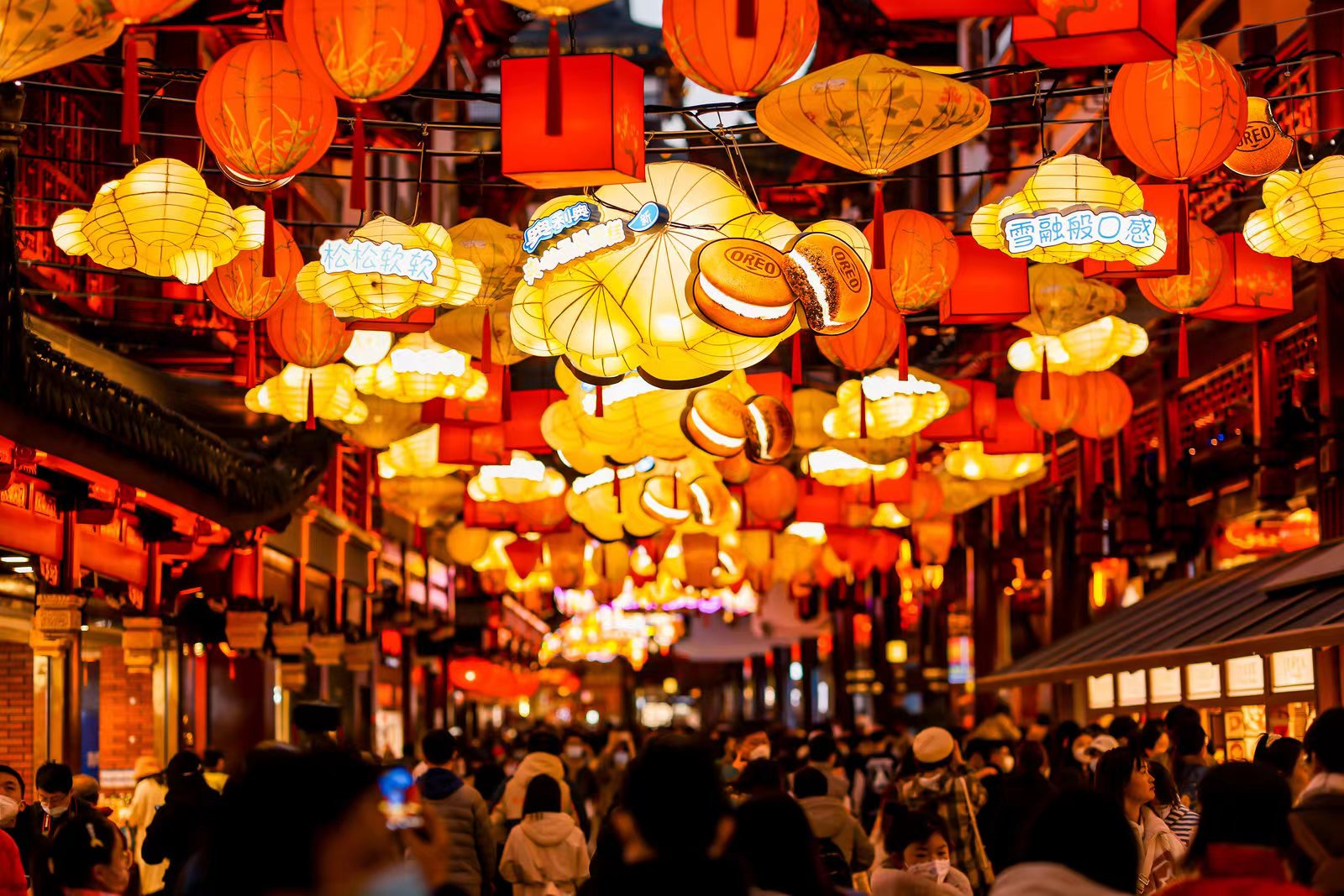The photograph captures a bustling nighttime scene in what appears to be a Chinatown or an Asian city district. The vibrant street is lined symmetrically with various businesses on both sides, bathed in a palette of deep oranges, yellows, and reds. Suspended above the street are dozens of brightly lit paper lanterns of different shapes, including flattened globes and boxes. Many of these lanterns feature intricate designs and Chinese or Japanese characters. Dominating the visual are several lanterns advertising Oreo cookies, with a specific mention of an orange variant with white cream filling. The streets below are teeming with people, many of whom are wearing face masks, hinting at contemporary times. The faces visible in the crowd suggest an Asian demographic, reinforcing the cultural ambience of the area. The overall aesthetic is a vivid, immersive snapshot of a lively Asian market street.